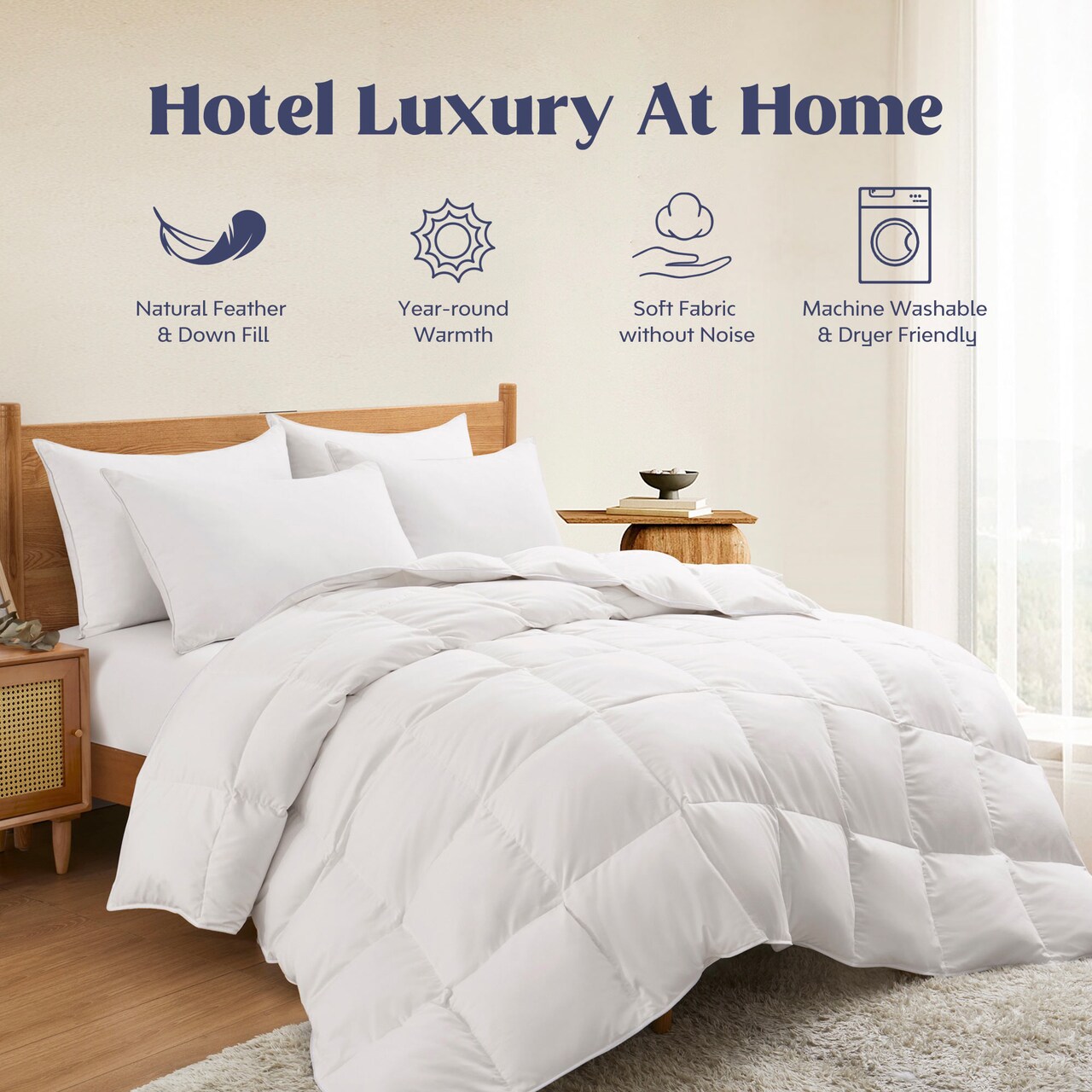The advertisement image, likely from a magazine, prominently features at the top the bold blue text "Hotel Luxury at Home." Below the text are four icons with descriptive phrases: a feather symbol labeled "Natural Feather and Down Fill," a sun symbol marked "Year-Round Warmth," a hand holding a cloud or nose with the text "Soft Fabric Without Noise," and a washing machine icon reading "Machine Washable and Dryer Friendly." The background is an inviting scene of a pristine white quilt and four matching pillows adorned on a bed with a brown wooden frame. Accompanying the bed are side tables crafted from similar brown wood, set within a room that exudes cleanliness with its white walls, white curtains, and ample natural light streaming in. A cream-colored rug rests atop a wooden floor, adding to the serene and luxurious ambiance.